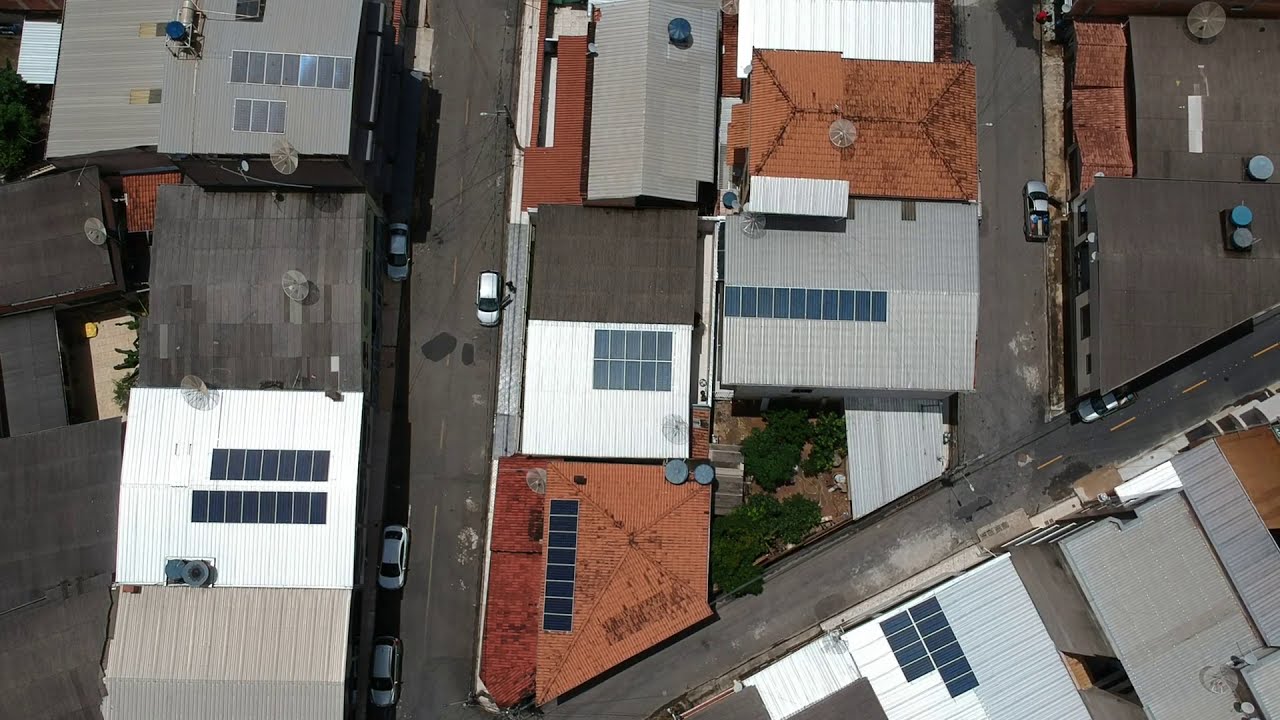This overhead drone shot provides a detailed bird's eye view of a densely built urban residential community. The image captures a network of city streets, including a horizontal two-lane street intersecting with a vertical one at the center, and a diagonal road running through the composition. The buildings, primarily apartment complexes up to four stories tall, showcase a variety of roof types, including red terracotta tiles, metal gray shingles, and darker gray roofs. Many roofs feature solar panels and satellite dishes, with some also housing exhaust fans. The neighborhood appears well-maintained, with clean and swept streets dotted with parked European-style cars. The architectural layout, combined with the array of rooftop details and the distinct European vehicles, adds rich texture to this vibrant urban tapestry.